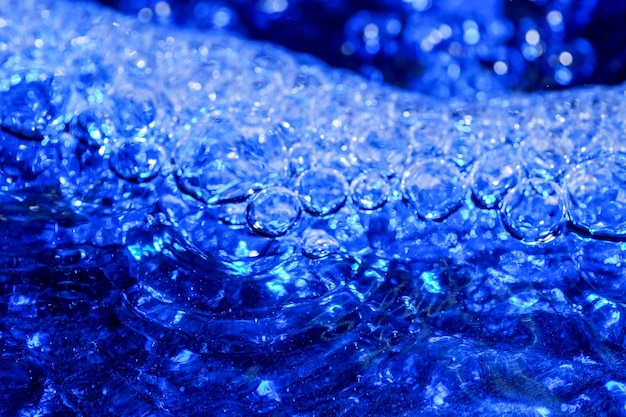This image features a horizontal, rectangular close-up view dominated by shades of blue. It depicts a multitude of wobbly, spherical, and largely see-through globes that resemble raindrops or bubbles. These globes vary in size and exhibit a somewhat distorted shape with a reflective, shiny surface. The top part of the image is filled with these spherical bubbles, which appear solid and densely packed, while the bottom half showcases a shiny, almost translucent blue material with lighter specks and an arc-like ripple pattern slightly left of the center. The background includes additional out-of-focus blue and white shiny areas, enhancing the image's overall wet, glistening aesthetic.